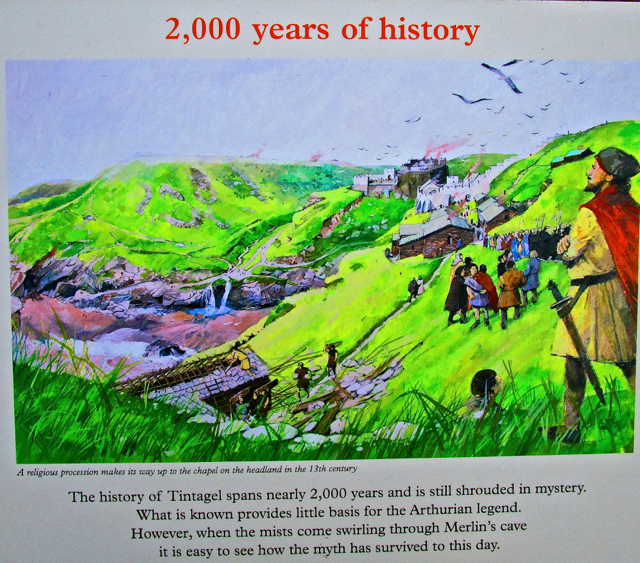This is an image from a history book featuring a detailed water paint drawing on a dark gray background. The page is titled in large red letters, "2,000 Years of History." The artwork depicts a vivid scene of green rolling hills with a small community scattered across them. Central to the image is a river cascading down into a small blue waterfall, which interestingly turns red upon hitting the ground. Sporadically placed buildings, including a green one on the left and a gray one to the right with red smoke emerging, embellish the landscape.

A chapel with a brown facade and white sloped roof sits amidst stone steps and walkways. A procession of people trails from the right side of the image, with some individuals congregating mid-hill, scaling up to the chapel’s vicinity. Birds uniquely fly backwards in the background sky, adding an ethereal touch.

On the far right stands a man, donning a yellow suit with a black belt securing a sword, a red cape cascades down his back, and he is topped with a gray hat. His contemplative gaze is directed to the left. At the bottom left corner, another man in yellow appears to be repairing a roof devoid of shingles.

Below the image, black text on the gray background provides historical context: "A religious procession makes its way up to the chapel on the headland in the 13th century. The history of Tintagel spans nearly 2,000 years and is still shrouded in mystery. What is known provides little basis for the Arthurian legend. However, when the mists come swirling through Merlin's cave, it is easy to see how the myth has survived to this day."